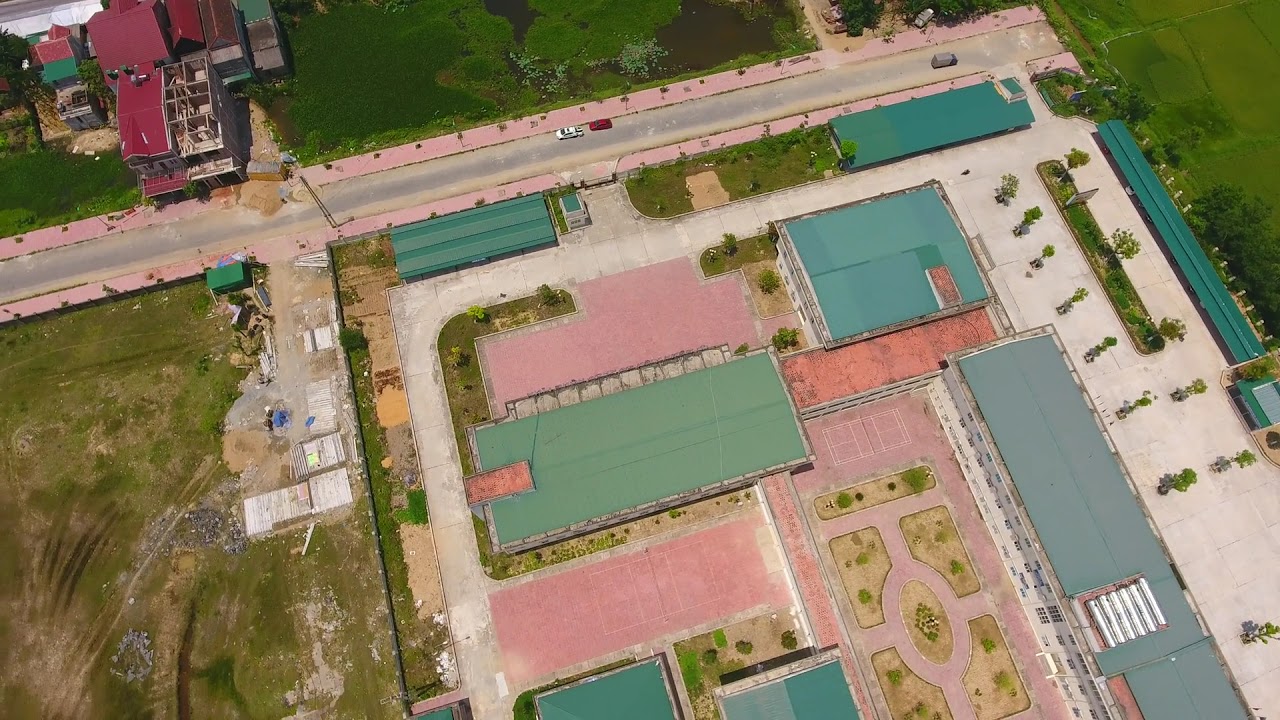This is an aerial, top-down view of a sizable complex that could be a school or business center. The complex is primarily situated to the right of the center of the image, with numerous buildings featuring mostly green, slate-colored roofs and one distinctive red roof. Between the buildings, there are concrete walkways, and in the middle, a courtyard with a decorative oval garden containing grass and possibly trees. This central courtyard also has walkways extending from both the top and bottom.

Towards the left of the image, there's a large grassy field and signs of construction activity. Surrounding the main complex area is an additional road or walkway lined with trees. At the far right, a large parking lot with areas of gray cement interspersed with planted trees can be seen. 

In the top portion of the image, a diagonal road runs from the near-right corner to the left middle. This road, which has cars on it, underscores the perspectives of this expansive urban block complex. Roofs of more buildings and additional trees are visible across the street from the complex.